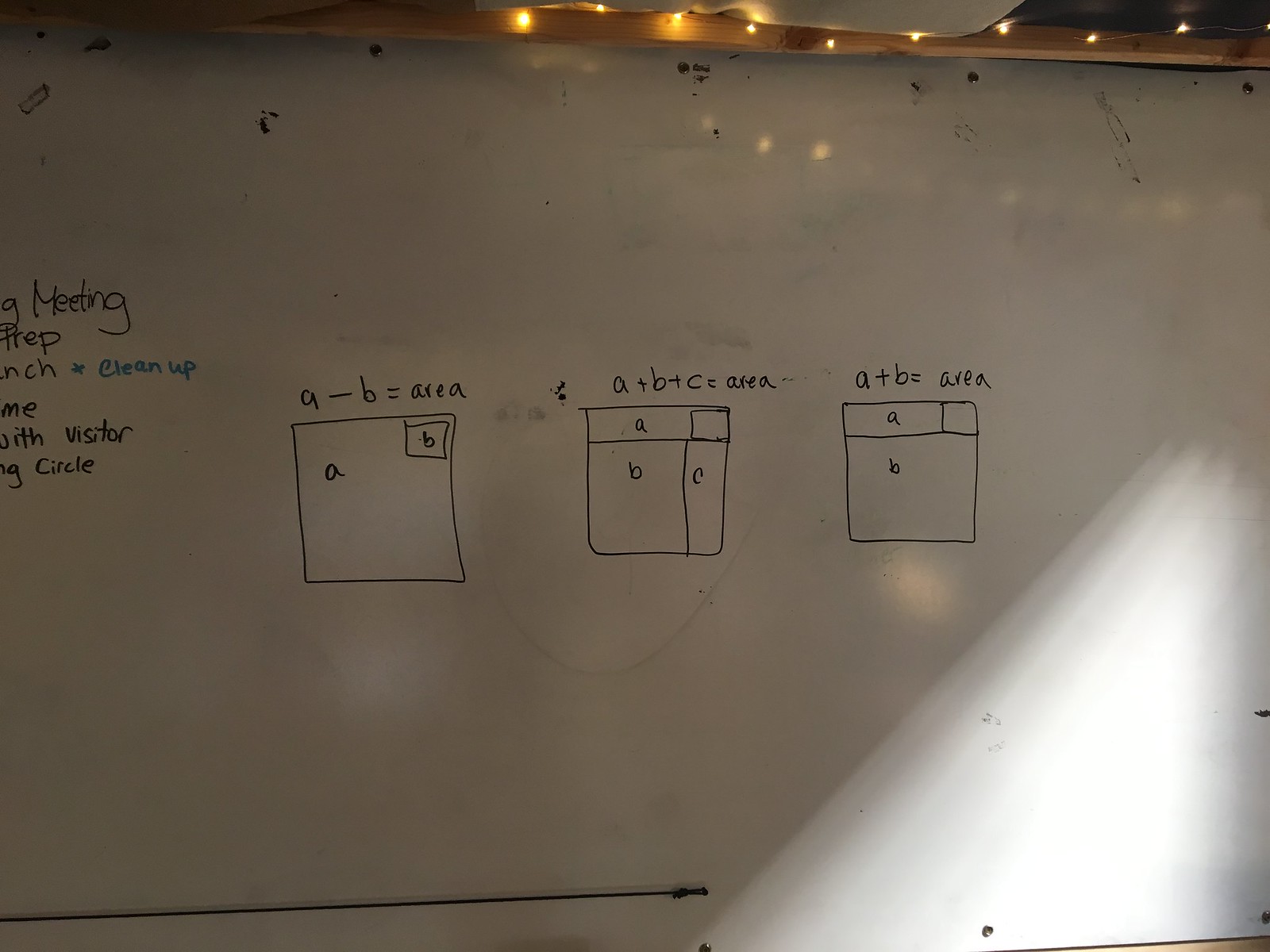The image showcases an extensive whiteboard that spans the entire surface. Written with a black marker, the board features various geometric formulas related to the area of squares. There are three distinct drawings of a large square, each labeled "A," used to illustrate these formulas.

1. **First Drawing:** The large square "A" contains a smaller square labeled "B" positioned in the upper right corner. Above this drawing is the formula "A - B = Area," indicating the area of the large square minus the area of the smaller square.

2. **Second Drawing:** The same large square "A" is now divided into three sections, labeled A, B, and C. The formula "A + B + C = Area" is written above, suggesting that the combined areas of these three sections equal the area of the large square.

3. **Third Drawing:** The final version of the large square "A" is divided into two sections, marked A and B. The accompanying formula "A + B = Area" implies that the sum of these two areas constitutes the entire area of the large square.

Overall, the whiteboard presents a progression of equations and illustrations to visually demonstrate different ways to conceive the area of a square and its components.